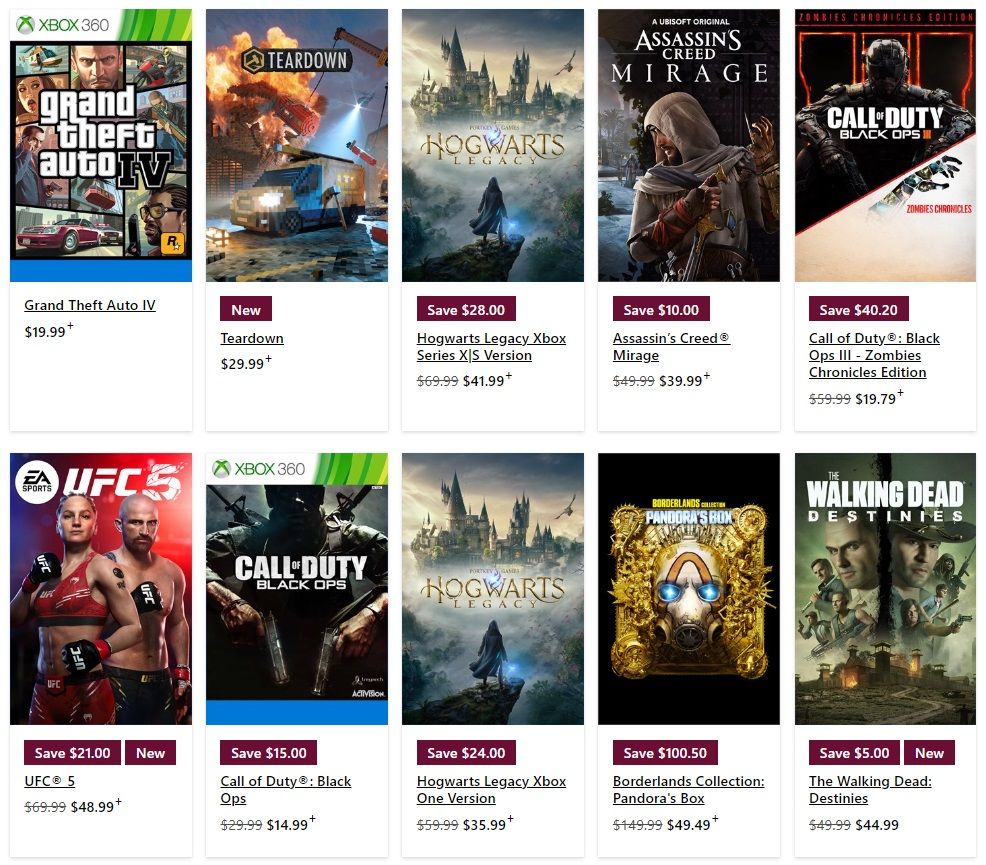The image is a structured grid comprising five long rectangles aligned vertically from top to bottom, enclosed within a square. Each rectangle contains two columns of video games, arranged horizontally from left to right. 

In the first row, the left column features "Grand Theft Auto," an Xbox 360 game, while the right column displays "Teardown." The second row has "Hogwarts Legacy" on the left and "Assassin's Creed Mirage" on the right. In the third row, "Call of Duty: Black Ops" is shown on the left, paired with another "Call of Duty: Black Ops" on the right column. The fourth row presents "Borderlands Collection: Pandora's Box" on the left and "Walking Dead: Destinies" on the right. Lastly, the fifth row includes "UFC 5," a boxing game, and another "Call of Duty: Black Ops."

Each game cover is visible, providing a visual context for the titles. Beneath each game cover, there is a "Save" button, allowing users to save the game. Notably, the first and last games in the bottom row possess an additional "New" button beside the "Save" button. However, the second game in the top row only features a "New" button, lacking the "Save" option.